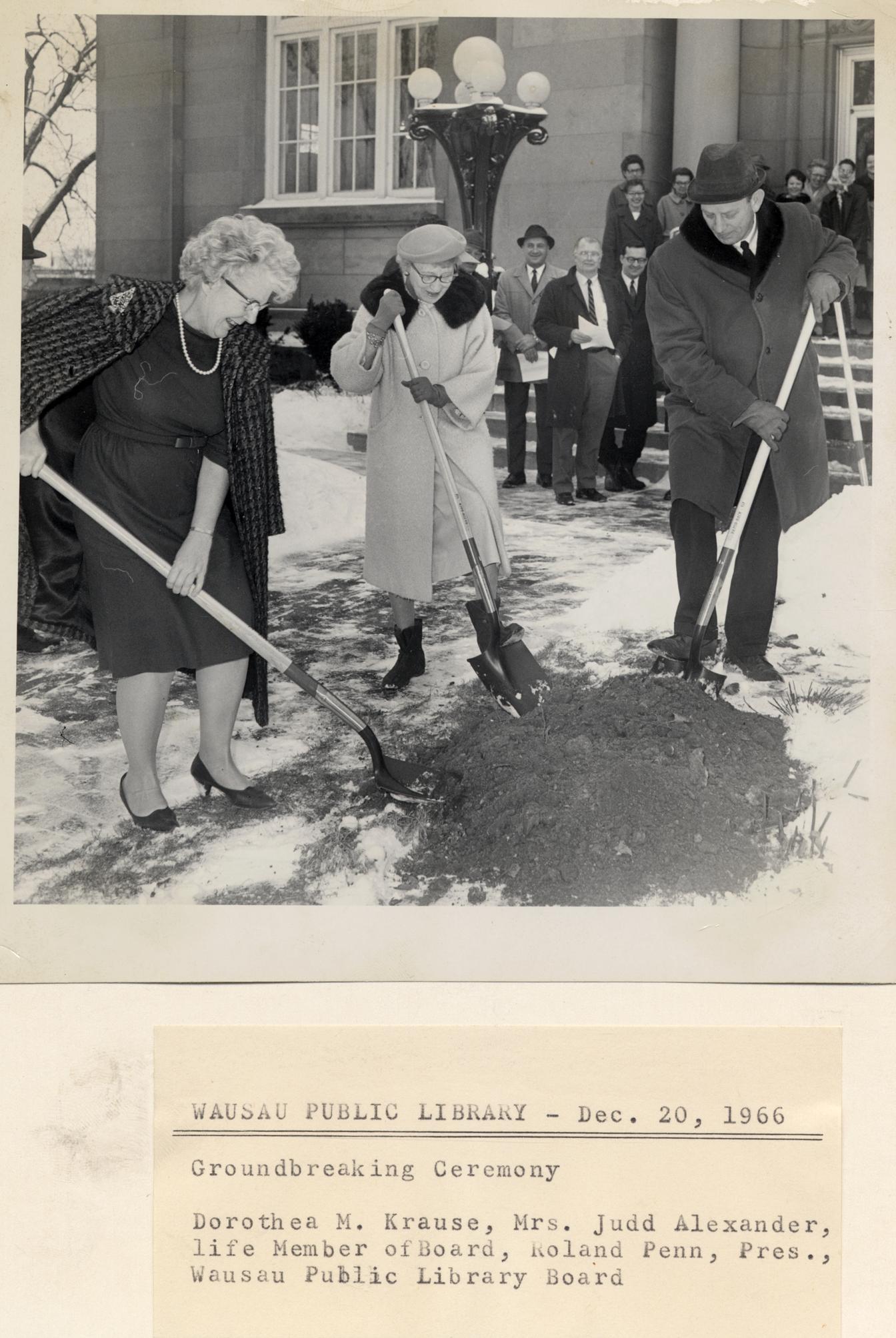A black and white vintage photograph from December 20, 1966, captures a significant moment in the history of the Wausau Public Library. The scene depicts a groundbreaking ceremony with three distinguished individuals: Dorothy M. Krause, Ms. Judd Alexander—a life member of the board—and Roland Penn, President of the Wausau Public Library Board. They are gathered around a pile of dirt, shovels in hand, poised to make the first dig to mark the beginning of a new library construction. The trio is dressed warmly in heavy winter coats and hats, against a backdrop of snow, reflecting the cold season. Dorothy Krause, on the left, is an elderly lady wearing a dress with heels. Ms. Judd Alexander, situated in the middle, dons a long, light-colored coat and black shoes. To her right, Roland Penn is dressed in a suit and heavy coat. Behind them, an engaged audience of men and women in suits and dresses stands on the steps of a building, likely the library-to-be. A lantern post is visible in the background, adding to the historic ambiance of this celebratory and community-focused event.